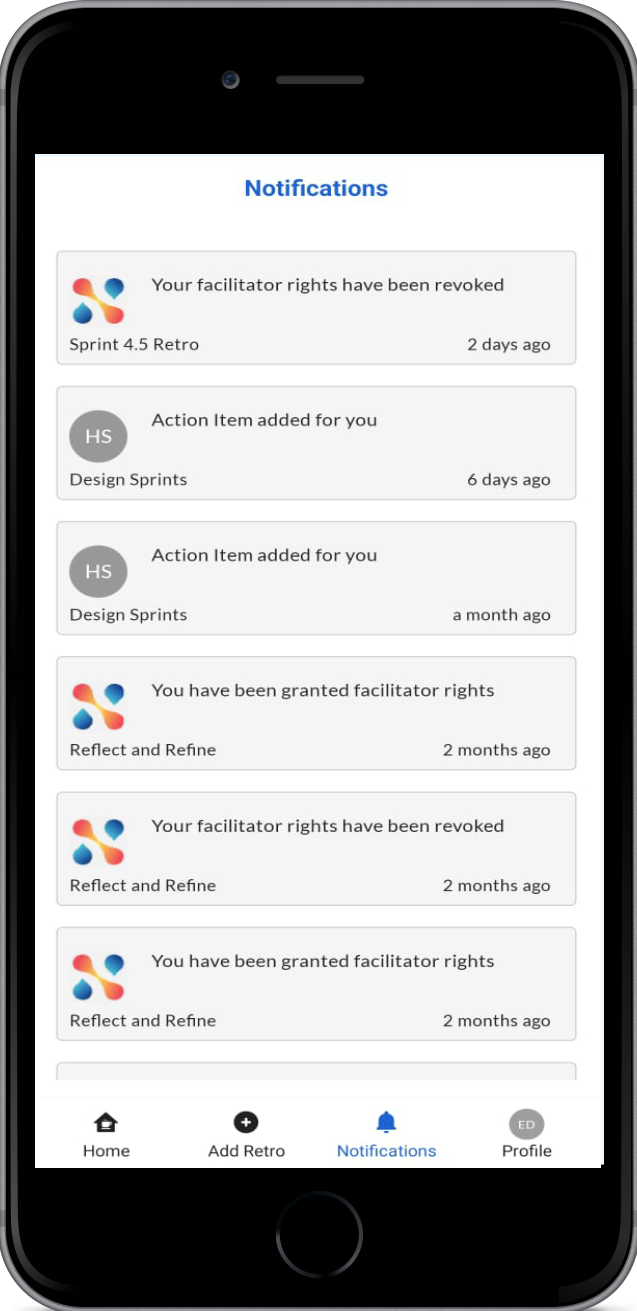The image displays a black cell phone against a white background. At the top edge of the phone's screen, the word "Notifications" is prominently displayed in bright blue font. Below this, there are several horizontal rectangular sections on a light gray backdrop. 

The first section features a logo on the left, colored blue and orange. In black text, it states, "Your facilitator rights have been revoked." Beneath the logo, the text reads "Sprint 4.5 Retro," and on the right side, it indicates "two days ago."

The second section includes a gray circular icon with the white initials "HS." The text reads, "Action item added for you." Below this, it says "Design Sprints," and on the right side, it notes "six days ago."

The third section is similar to the second, with the same gray circular icon and initials "HS." It reads, "Action item added for you," followed by "Design Sprints," and on the right side, it mentions "a month ago."

The last three sections each have the same blue and orange logo on the left. They read "Reflect and Refine" with the right side stating "two months ago." The first of these states, "You have been granted facilitator rights." The second reads, "Your facilitator rights have been revoked." The third says, "You have been granted facilitator rights."

At the bottom of the phone screen, there are icons labeled "Home," "Add Retros," "Notifications," and "Profile." The "Notifications" icon and label are highlighted in blue.